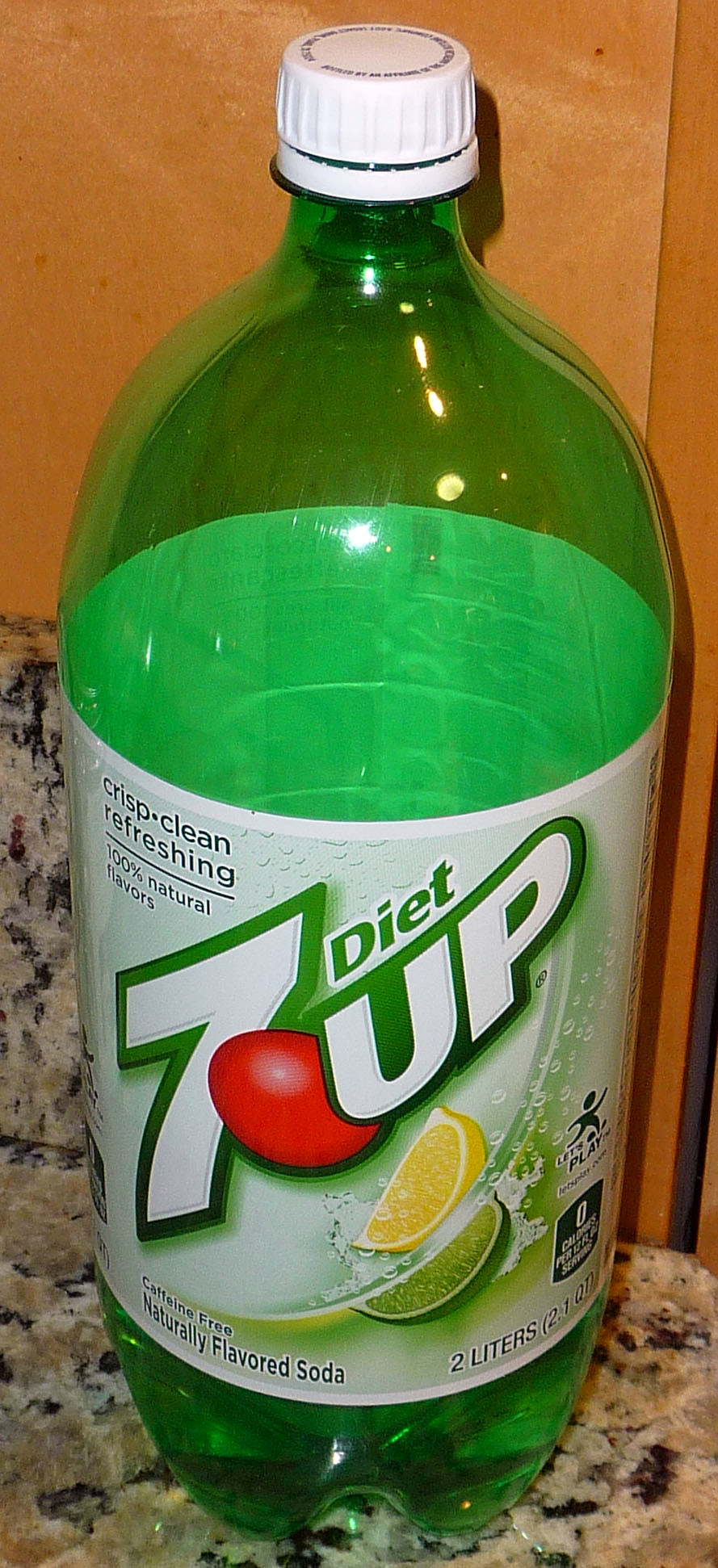This close-up photograph showcases a two-liter bottle of Diet 7-Up on a marble kitchen bench, in front of a medium oak-colored wooden wall. The bottle is green with a white cap and white label. Its green label features "Diet 7-Up" written in large, angled text, with a prominent '7' pointing to the left and 'Up' oriented towards the right. Beneath the logo, there is a red egg-shaped graphic, along with images of a lemon and lime.

The label's top-left corner displays the words "Crisp, Clean, Refreshing" followed by "100% Natural Flavors." Further details on the bottom-left of the label include "Caffeine-Free, Naturally Flavored Soda" and indicate the bottle size as "2 Liters (2.1 Quarts)" along with "Zero Calories per serving." There's also a small logo of a person with the words "Let's Play" above additional text near this information.

The bottle appears empty or contains very little liquid, which is difficult to discern from the provided angle. The marble countertop, described as brown, white, grey, and black-spotted, slightly frames the image, reinforcing the kitchen setting.